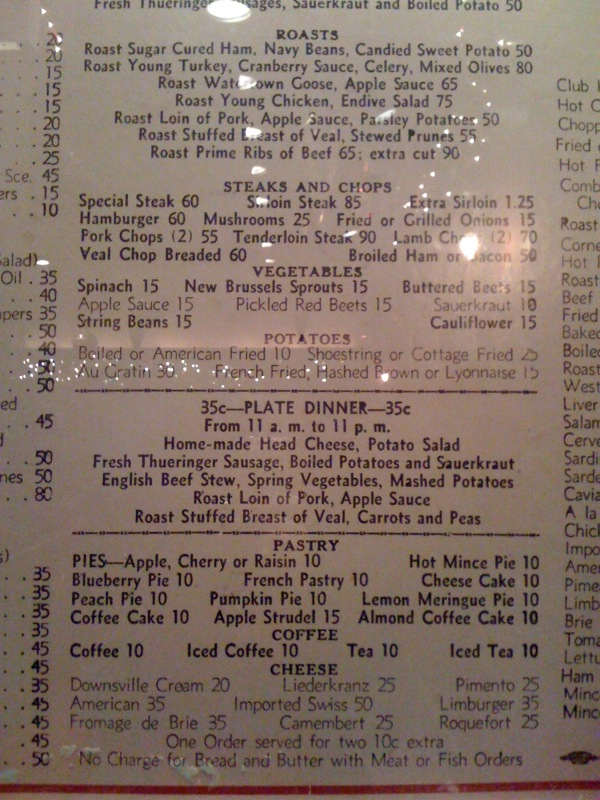This photograph captures a vintage menu from a restaurant, offering a glimpse into the culinary options and pricing of a bygone era. The menu prominently features a section titled "Roasts," which includes a tempting variety of dishes such as cured ham, navy beans, roast turkey, roast water tongue goose, roast young chicken, roast loin of pork, and roast stuffed breast of veal. Below this, the menu transitions to "Steaks and Chops," featuring options like special steak, sirloin steak, and extra sirloin.

Further down, there is a "Vegetables" section listing sides like spinach and Brussels sprouts. The "Plate Dinner" section announces a complete meal available for just 35 cents, served from 11 a.m. to 11 p.m. Notably, a special steak costs a mere 60 cents and a sirloin steak is priced at 85 cents, illustrating the affordability of meals at the time.

The photograph appears to have a glare, perhaps from ambient lighting or reflective surfaces, indicating that the menu might have been preserved under glass. This nostalgic artifact offers a fascinating snapshot of historical dining experiences and economical prices, framed by the ambiance of the restaurant in which it was photographed.